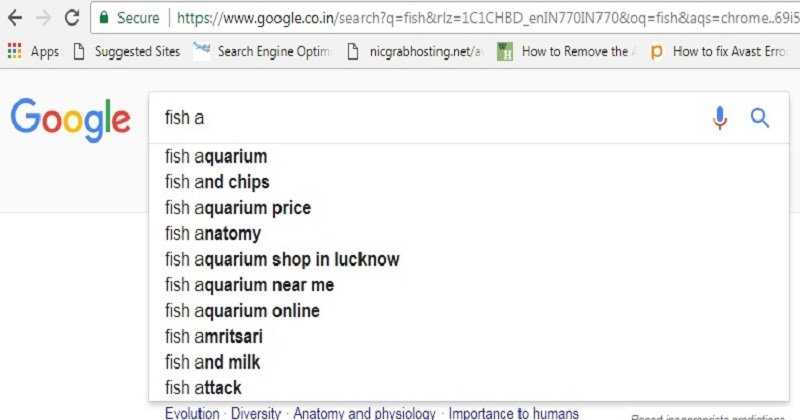The image showcases a screenshot of a Google search page. The user has begun typing in the search bar, starting with "www.google.co.in" followed by additional, likely mistyped characters. At the top-left corner, the Google logo is visible, displaying its iconic colorful letters.

In the search bar, the partially typed query "fish a" is seen. As the user begins to type, Google's autocomplete suggestions appear in a dropdown menu below the search bar. The suggested search terms include:
1. Fish aquarium
2. Fish and chips
3. Fish aquarium price
4. Fish anatomy
5. Fish aquarium shop in Lucknow
6. Fish aquarium near me
7. Fish aquarium online
8. Fish Amrit
9. Fish and milk
10. Fish attack

These suggestions are listed within a rectangular box that appears below the search bar. In the same rectangle, to the right of the "fish a" typed query, there is a microphone icon indicating the option for voice search. Below this, a magnifying glass icon is seen, signifying the search button.

At the bottom of the screenshot, there are visible tabs or headings, one of which reads "Evolution Diversity Anatomy and Physiology Important to Humans", hinting at related search topics.

Overall, the image captures a typical moment of a user beginning a search on Google, highlighting the platform's autocomplete feature and the diverse range of topics people commonly search for starting with "fish a".